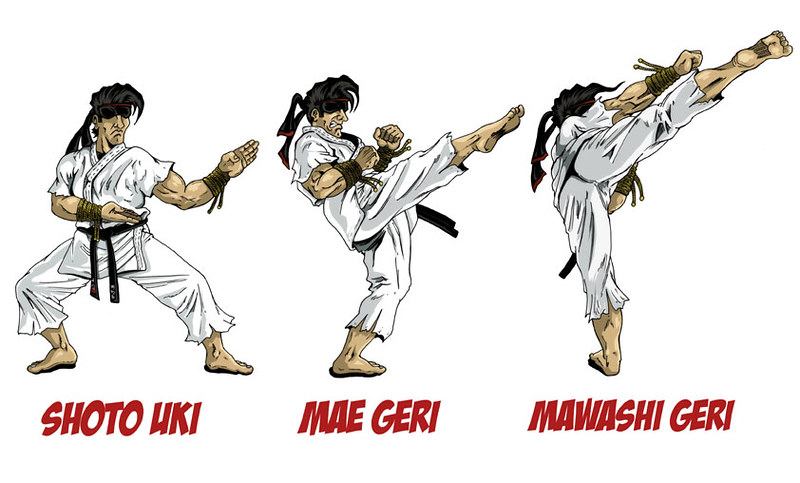The image features a cartoon character depicted in three different martial arts poses against a white background, showcasing various aspects of his skill. The character is dressed in a traditional white karate uniform with a black belt, black bandana tied around his head, and leather bracelets adorning his wrists, and he is barefoot.

In the first pose on the left, labeled "Shoto Yuki" in red lettering, the character faces forward with his legs spread wide and his body slightly squatted. His left arm is bent and raised outward at the elbow, while his right arm extends across the front of his body, poised for action. 

The middle pose, captioned "Mae Geri," presents a profile view of the character’s right side. Here, he strikes a high kick with his right leg fully extended forward. His fists are clenched and held close to his torso, and his facial expression shows determination with his teeth visible.

The final pose on the right, labeled "Mawashi Geri," is featured from a rear angle. The character balances on his left foot, with his torso bent forward and his right leg extended high into the air. The sole of his raised foot points upward, parallel to his arm, and the back of his head and the tied bandana are clearly visible.